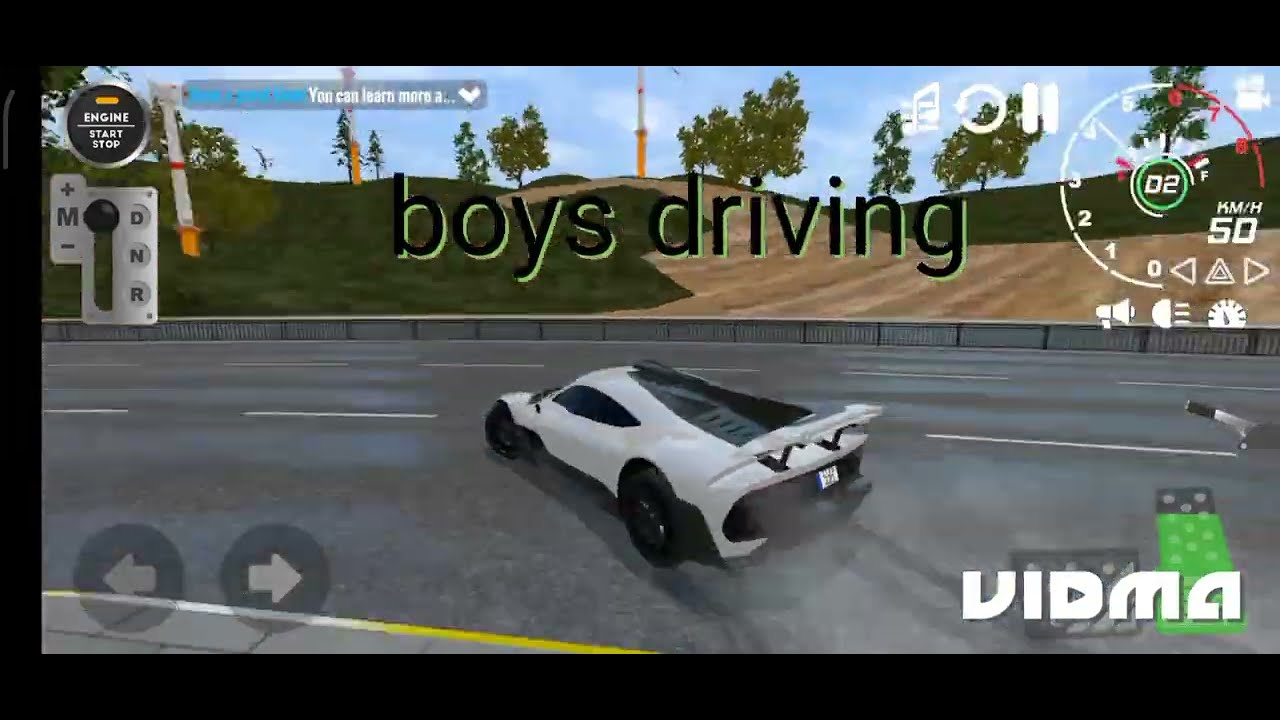The screenshot captures a detailed interface of a racing video game featuring a sleek, white sports car, possibly a Supra, Lamborghini, or Ferrari. The car is maneuvering around a four-lane road with a yellow-striped pedestrian walking area and appears to be spinning out of control. The vehicle boasts black tires, a spoiler, and a low, aerodynamic profile.

The UI is replete with informative elements. Centered at the top of the screen, bold black text outlined in light green reads "Boys Driving." Thin black bars frame the top, bottom, and the left side of the screen. The bottom right corner displays a lit-up green accelerator pedal indicator, while a non-lit flatter rectangle on the left indicates the brake pedal. A watermark or logo labeled "Vidma" is visible above the pedal indicators.

Additional icons populate the top right corner: a tachometer extending up to 8,000 RPM with the red zone beginning at 6,000 RPM, a speedometer indicating 50 kilometers per hour, alongside symbols for a clock, microphone, and lights. The upper left corner features engine controls marked "Engine Start Stop" and a shifter display showing "D N R M" for driving modes. Blue text in this area, blending into the background, reads "You can learn more A." A conspicuous black circle with a white check mark sits near this text.

The gaming environment includes picturesque elements such as windmills, green grass, and trees scattered in the background. The overall design offers an immersive and detailed racing experience, emphasizing both aesthetic appeal and functional UI elements.